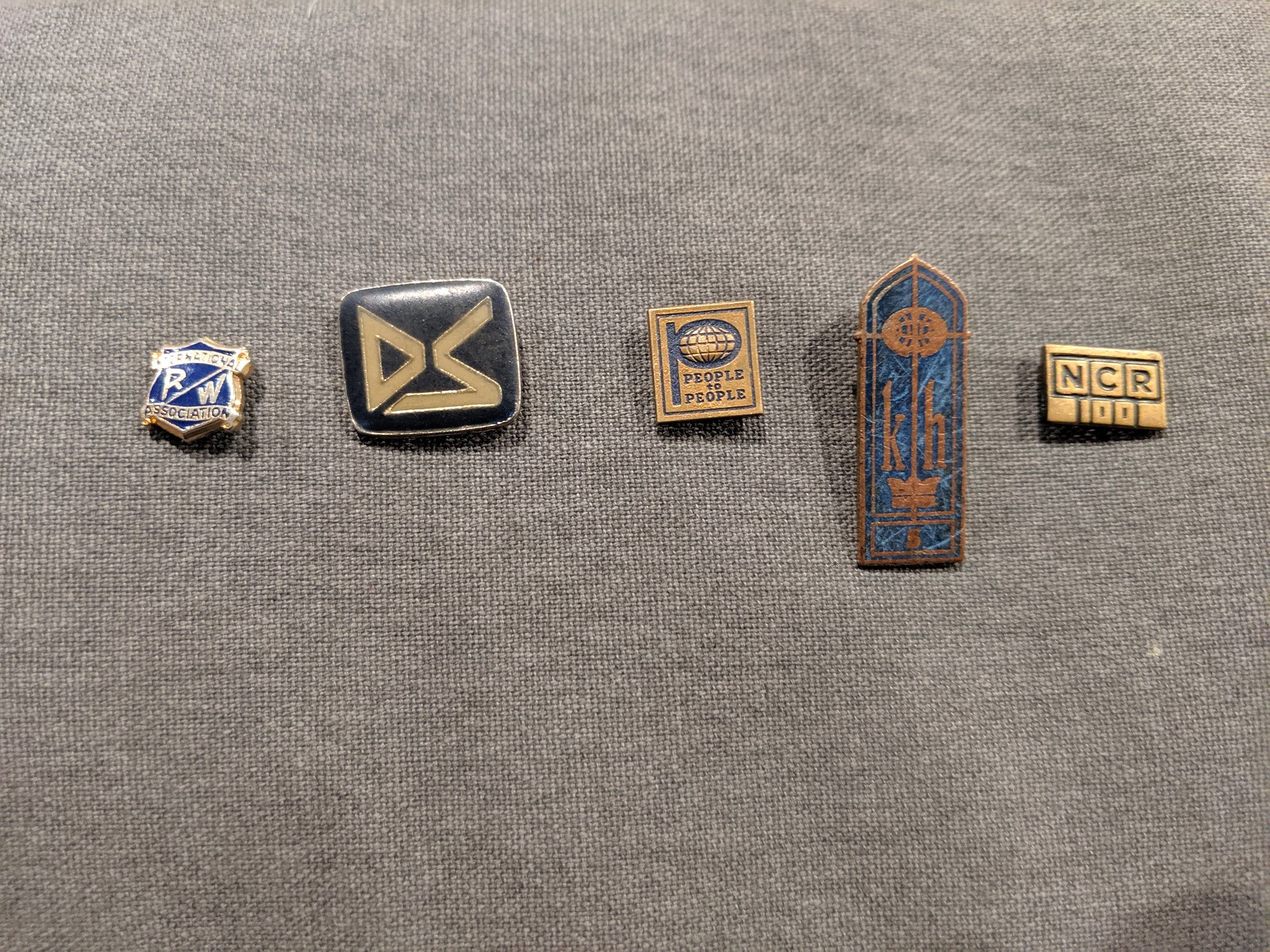The photograph showcases five distinct lapel pins, all varying in shape and size, elegantly arranged on a grayish-brown canvas fabric background with noticeable wrinkles particularly in the top-right and bottom-right sections. 

From left to right:
1. A dark blue shield-shaped pin with a gold border and the initials "RW" prominently displayed.
2. A black rounded square pin bearing gold symbols, specifically the letters "DS" in a tan color.
3. A square pin featuring the words "People to People," adorned with a blue "P" and a gold globe emblem.
4. A pin shaped like a window, colored in blue and tan, showcasing a crown with the letters "KH" on the front.
5. A light brown rectangular pin, marked with the letters "NCR" in black.

A subtle shadow, likely cast by the person taking the picture, adds depth to the composition. This precise array and the distinct details of each pin illustrate a collection that is both eclectic and meticulously curated.